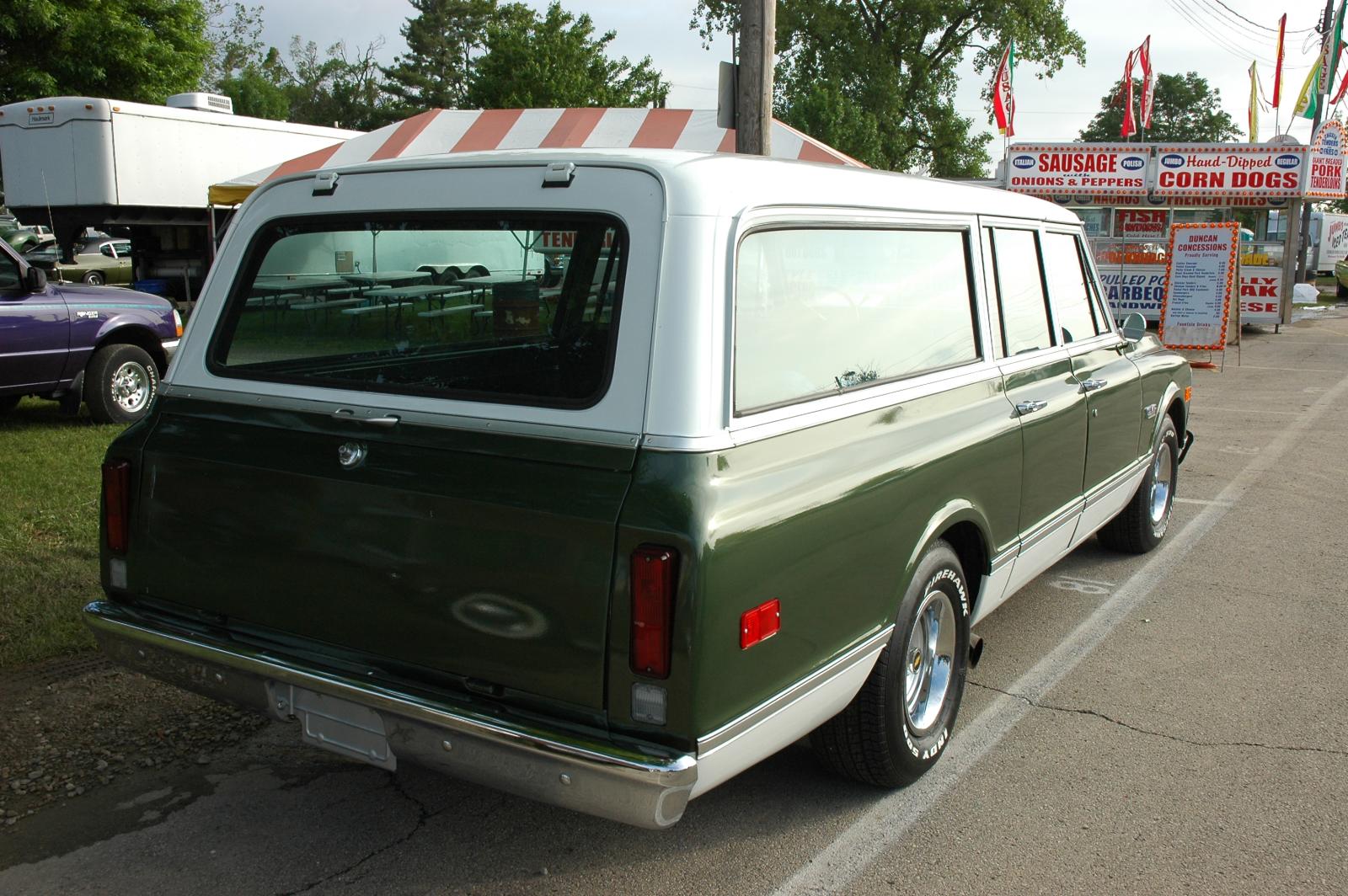The image depicts a very old-fashioned, well-maintained green and white station wagon, which looks like an old Suburban, parked on a driveway at a carnival. The car, sporting brand new tires, has a white top, green middle, and white bottom, complemented by black tires and silver rims. To the left of the station wagon, there is a grassy area with a blue vehicle visible in the distance. Adjacent to the car is a prominent food stand advertising sausage, hand-dipped corndogs, onions, and peppers, with a striking red and white striped pop-up tent above it. The stand is adorned with colorful red, yellow, and green flags. Additionally, there is an A-frame pricing sign on the sidewalk and a trailer with an air conditioner in the background to the left, in front of which a small pickup truck with silver rims is parked. The scene is framed by distant trees and a bit of sky, completing the bustling carnival atmosphere.